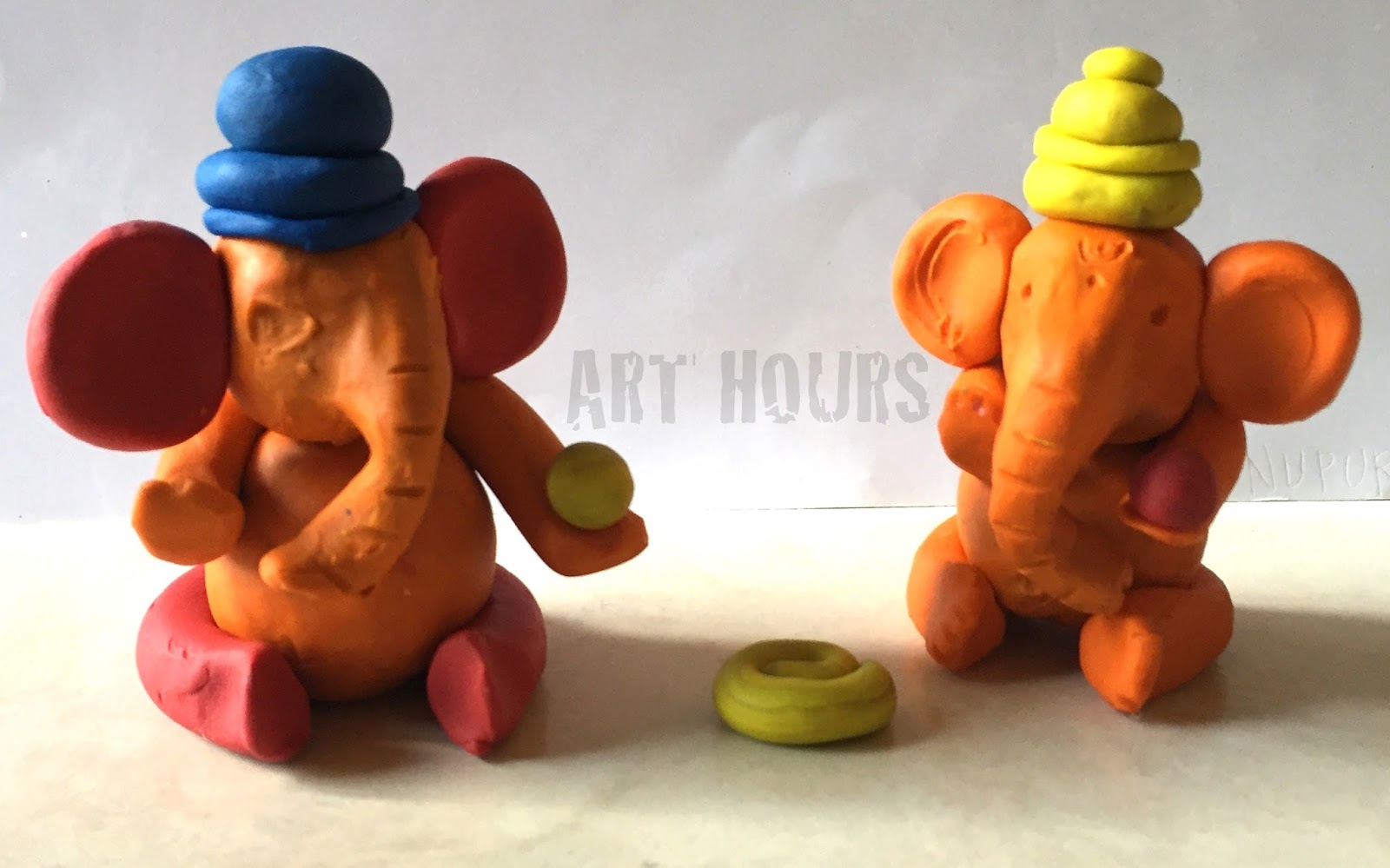This detailed photograph showcases a clay art project against a crumpled white background with a faint gray watermark reading "Art Hours" and "N-U-P-U-R" in the bottom right corner. The scene is set on a pale tan or yellow table, featuring two striking orange elephants crafted from polymer clay. These figurines are seated, facing each other with expressive details. 

The elephant on the left side has a combination of red ears and legs and dons a circular blue hat. It holds a small yellow ball in one outstretched hand. The elephant on the right mirrors its counterpart in color but has orange ears and legs, with its arms crossed, adorned with a tall yellow hat. A notable detail is the small yellow, rolled-up piece of clay resembling a cinnamon roll or croissant situated between them, adding a whimsical touch to this charming scene.